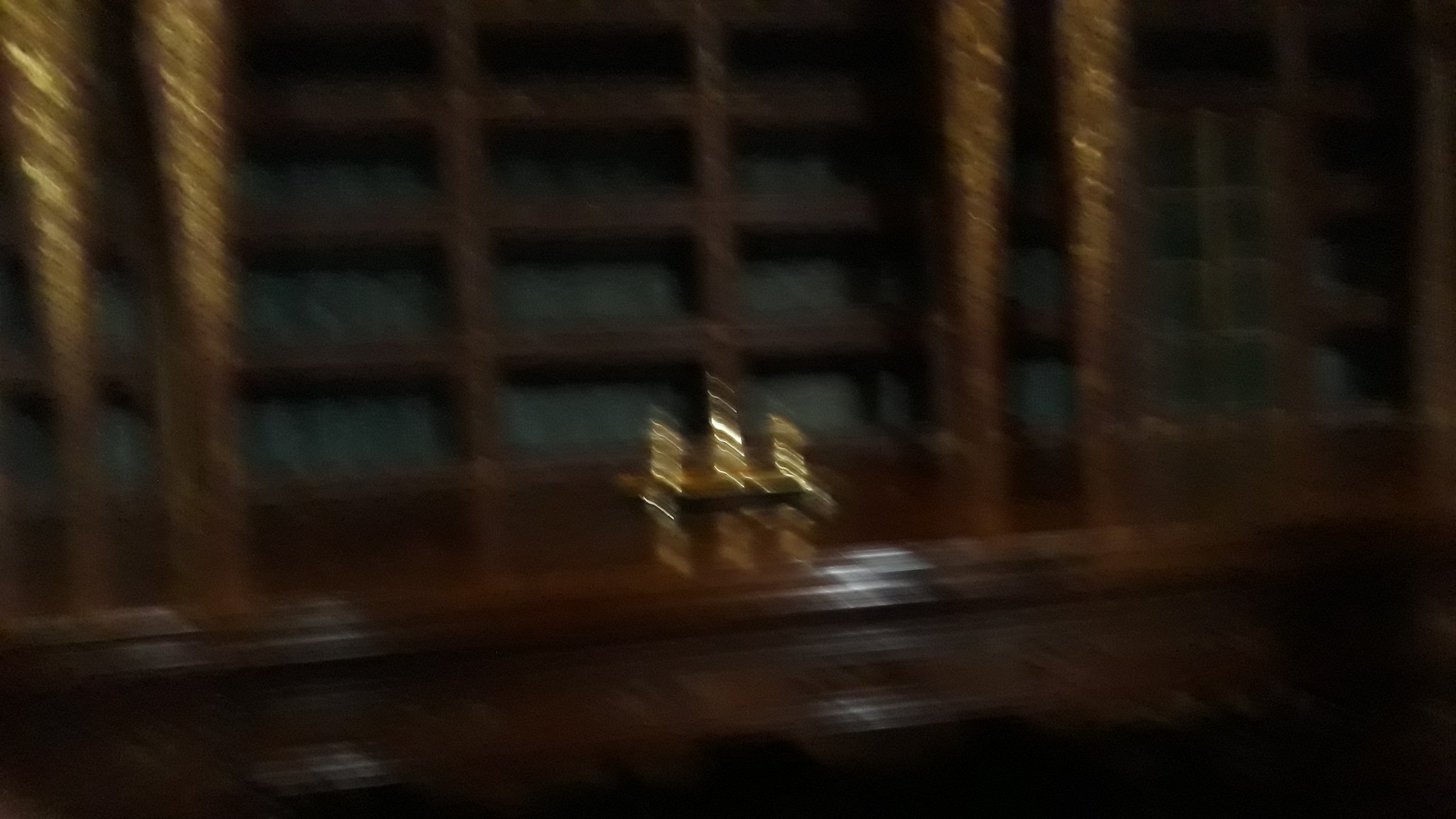A slightly blurry photograph captures a large wooden table that exudes a warm, mid-toned hue, blending shades of chocolate and caramel brown. Atop the table rests a golden object, though the image's lack of sharpness makes it difficult to discern its precise nature. Flanking the table are bookcases crafted from the same rich wood, enhancing the setting's cohesive aesthetic. Positioned on either side of the golden object, a pair of wooden columns adorned with delicate gold leaf designs add an element of sophistication. The table's front edge features intricately carved drawers, showcasing masterful craftsmanship, while light reflects softly off the surface, adding a gentle luminescence to the scene.